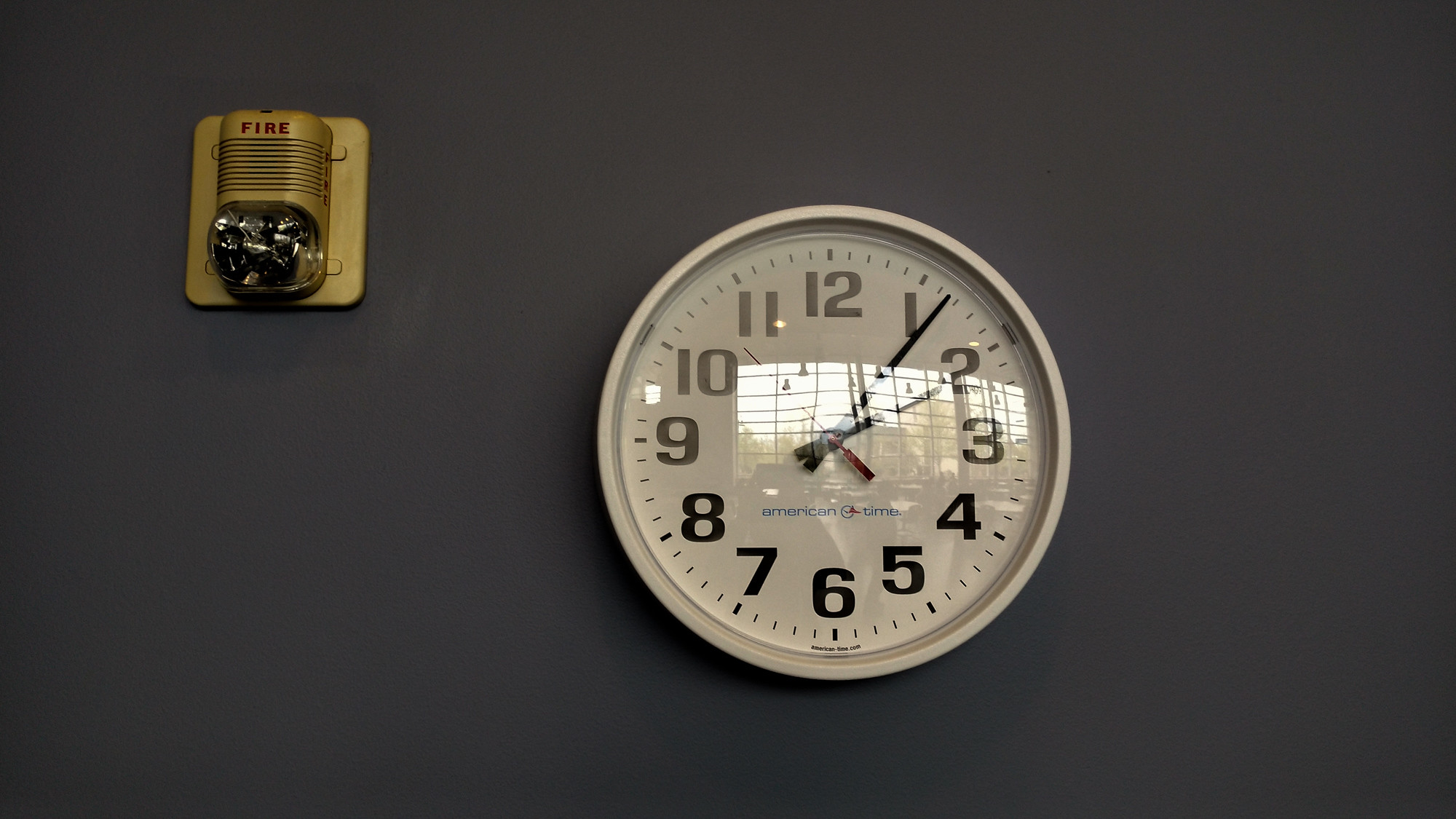In this photograph, a simple white clock with a white face and white border hangs on a dark gray wall. The clock features bold black numbers from 1 to 12 and thin black minute and hour hands, with a thin red seconds hand indicating the time, which is 2:06. Above the clock, in the upper left-hand corner, is a gold-colored fire alarm mounted on a square base with the word "FIRE" printed in red. The fire alarm has a design reminiscent of an old-fashioned microphone, with a speaker above a lens that likely flashes when the alarm is activated. The setting appears to be a school or public building, as suggested by the classic and functional style of both the clock and the fire alarm.